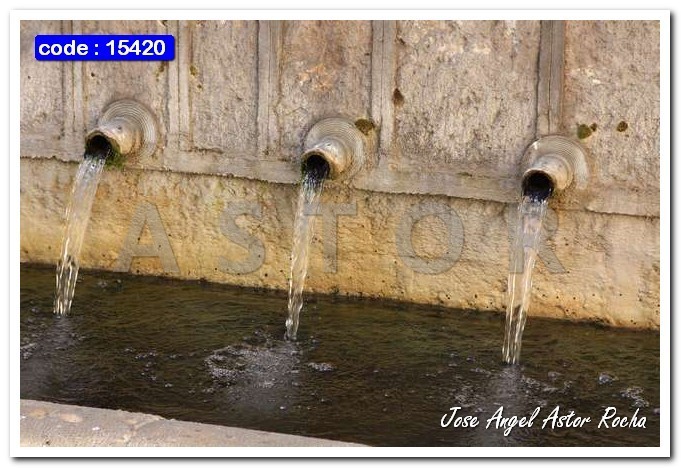This digital outdoor photograph captures a trio of drainage pipes embedded in a beige and light brown stone or concrete wall, positioned nearly equidistant from each other. These pipes are releasing water into a dark trough below, which is filled with water. The stone wall appears more green as it descends. A small section of the stone structure and a stone wall are visible to the left of the image. In the upper left corner, a blue rectangle bears the text "code 15420." Centered in the image is the word "ASTOR," and the bottom right corner is marked with the name "Jose Angel Astor Rocha" written in white cursive. The photograph is bordered in white.